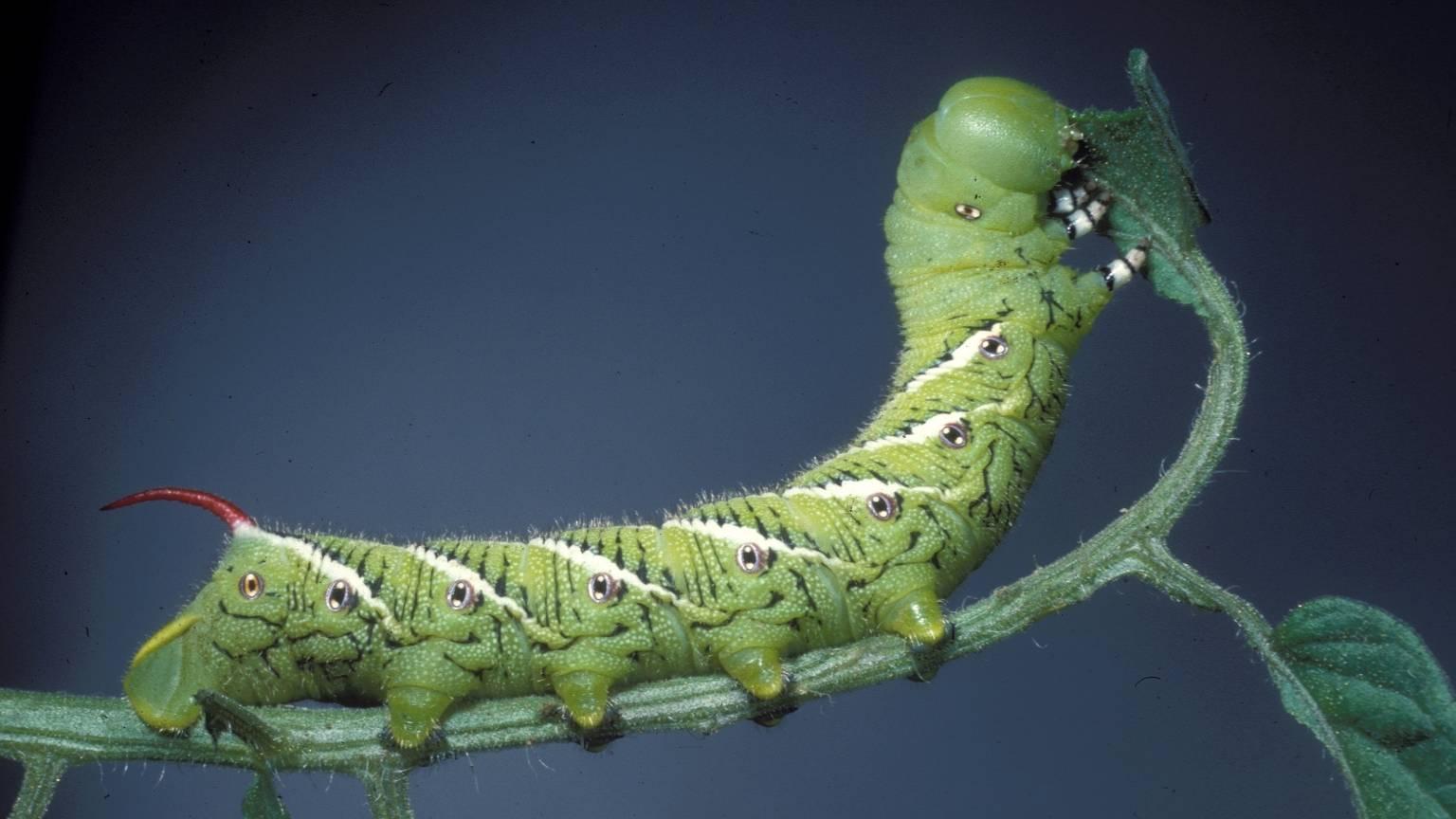This highly detailed close-up photograph captures a green caterpillar perched on a slender branch, avidly eating a leaf. The caterpillar, mostly light green in color, is adorned with black and white stripes along its sides, giving it a somewhat furry appearance. Adding to its distinctive look is a reddish-brown, slightly spiky tail at the end. The body of the caterpillar features a fascinating pattern of eye-like markings, accentuating a natural defense mechanism to deceive predators. Along the sides of its body, this pattern of eyes runs the entire length. Its feet, which appear to be ten in total though only five are visible, grasp onto the branch and surrounding leaves, while its tiny mouth works on the leaf, evident from numerous bite marks. The scene is set against a dark black backdrop, which contrasts sharply with the vibrant green of the caterpillar and the lush green leaves. The composition includes two leaves on the branch: one being actively gnawed on by the caterpillar, and the other hanging down from the branch, away from the insect.